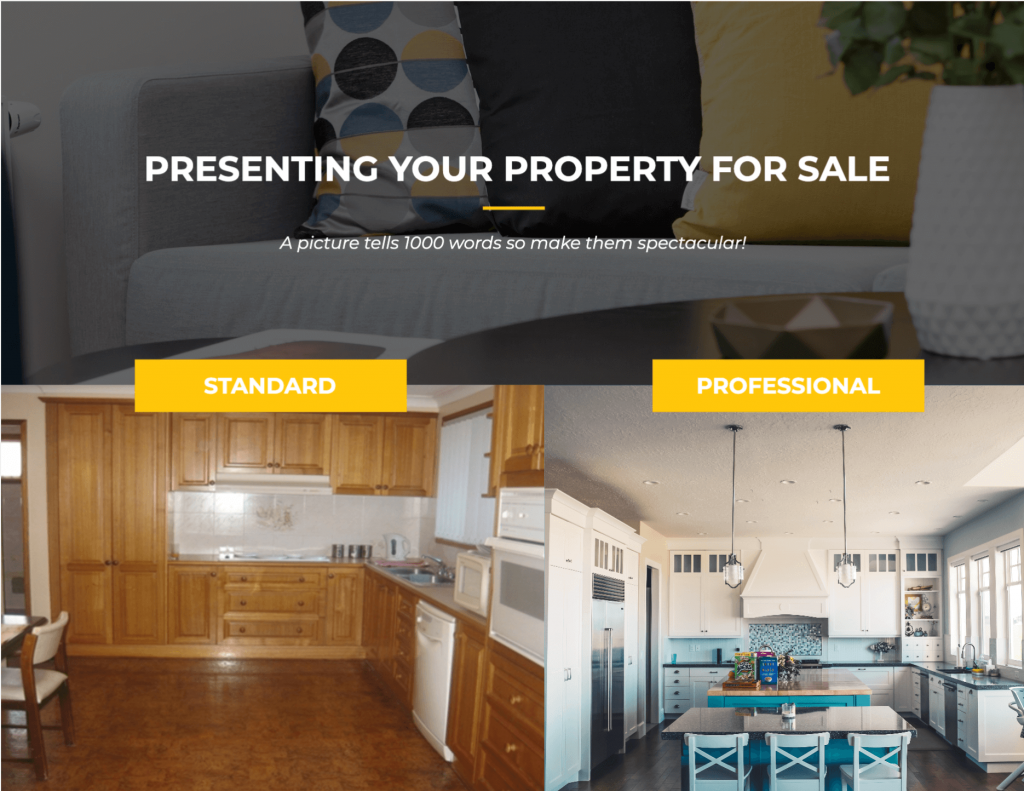This image is a screenshot of a professional real estate website, designed to showcase properties with high-quality photographs. The layout features three main images: the top half is dominated by a large picture of a stylish couch adorned with decorative pillows. Overlaying this image is bold white text that reads, "Presenting Your Property for Sale," followed by a thin yellow underline. Beneath this line, additional white text proclaims, "A picture tells 1,000 words. So make them spectacular."

Below this primary image, the bottom of the screenshot is divided into two smaller sections. On the left side, there is a standard photograph of a kitchen featuring mostly brown wooden cabinets and white appliances, creating a rather plain and conventional look. In contrast, the image on the right displays a bright and vibrant kitchen with a modern aesthetic, characterized by a white and teal color scheme with stainless steel appliances.